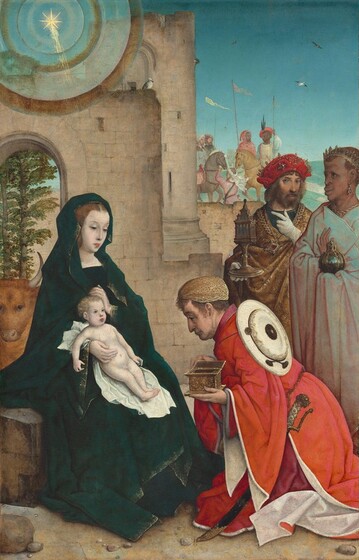In this detailed painting, an azure sky dominates the upper section, featuring a prominent star with concentric circles ranging from thin white to thicker brown bands. This heavenly symbol is positioned near the upper left corner, suggesting a scene of religious significance. The foreground is occupied by the Virgin Mary, adorned in a long black dress with a matching head covering, tenderly holding a naked baby Jesus on a white blanket. They are receiving three wise men, one of whom kneels before them, presenting an open box of gifts. This figure, with brown hair, a small brown hat, and an orange and white robe, displays white circles on their back, topped with a black circle.

Behind the kneeling visitor, another man is dressed in an off-white and brown robe, with an olive leaf headdress akin to Caesar's. He holds a spherical container resembling a pumpkin. The third wise man, sporting a beard and long brown hair, wears a gold-brown robe and a white glove, carrying an object that looks like a lamp. Further back, a man with a feathered turban and white robe stands, flanked by a person in a gold and orange cape, who faces away from the viewer. A brown and gray horse with a pinkish saddle appears beside them.

In the upper section of the scene, partially obstructing the view, is a stone castle with a visible archway revealing an evergreen tree and a brown cow or bull with prominent horns behind Mary and Jesus. Soldiers with spears and flags populate the right side of the background, adding a sense of vigilance and grandeur to this depiction of the nativity.